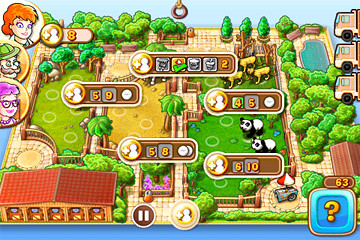The image depicts a vibrant, bustling garden or zoo set under a bright blue sky with a rainbow arching across the top. In the upper left corner, there is a circular icon featuring a character with orange hair, blue eyes, and pink lips. To the right of this icon is another circular icon in brown, flanked by a plus sign on the left and the number eight along with a silhouette of a person on the right. 

In the middle left section, a character wearing a green explorer's hat and sporting a large mustache stands out. To the far left, a person with striking pink hair, pink glasses, and a pink necklace is illustrated. 

At the very bottom of the image, there is a house with red-tiled roofing. The house has doors that appear to lead out to a tranquil river. The garden or zoo is vividly portrayed with various enclosures: the left enclosure houses animals while the right enclosure features black and white pandas amid lush greenery. 

Scattered throughout the image are symbols with numbers such as 59, 58, 6, 10, and 45, as well as icons in gray and orange with check marks inside them, notably one marked with the number two. Pink flowers add to the garden's vividness, and at the bottom right corner, there is a blue square featuring a yellow question mark, reminiscent of video game iconography.